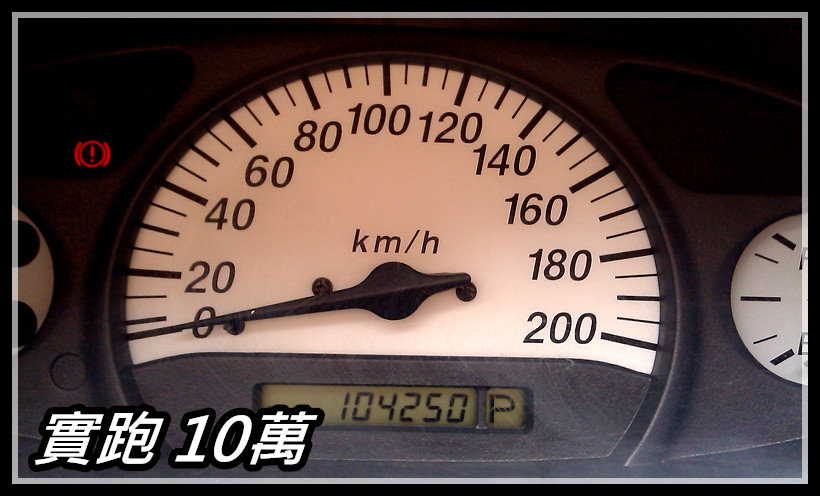A close-up image showcases a European-style car speedometer, measuring speed in kilometers per hour (km/h), ranging from 0 to 200 km/h. The speedometer's face is white with bold black numerals, each marked by a corresponding black line. The needle of the speedometer, also black, is positioned at 0 km/h, indicating the vehicle is stationary. Below the speedometer, an LED display shows the car's mileage, reading 104,250 miles, and another adjacent LED indicator reads 'P,' confirming the vehicle is in park. 

In the upper left section of the image, a vivid red warning light featuring an exclamation mark circumscribed by a circle is illuminated, suggesting an issue requiring engine inspection. On the right, part of the fuel gauge is visible, sharing the white-faced design with black demarcations. Additionally, the bottom left corner of the photo contains Japanese characters and the number '10,' embossed clearly.